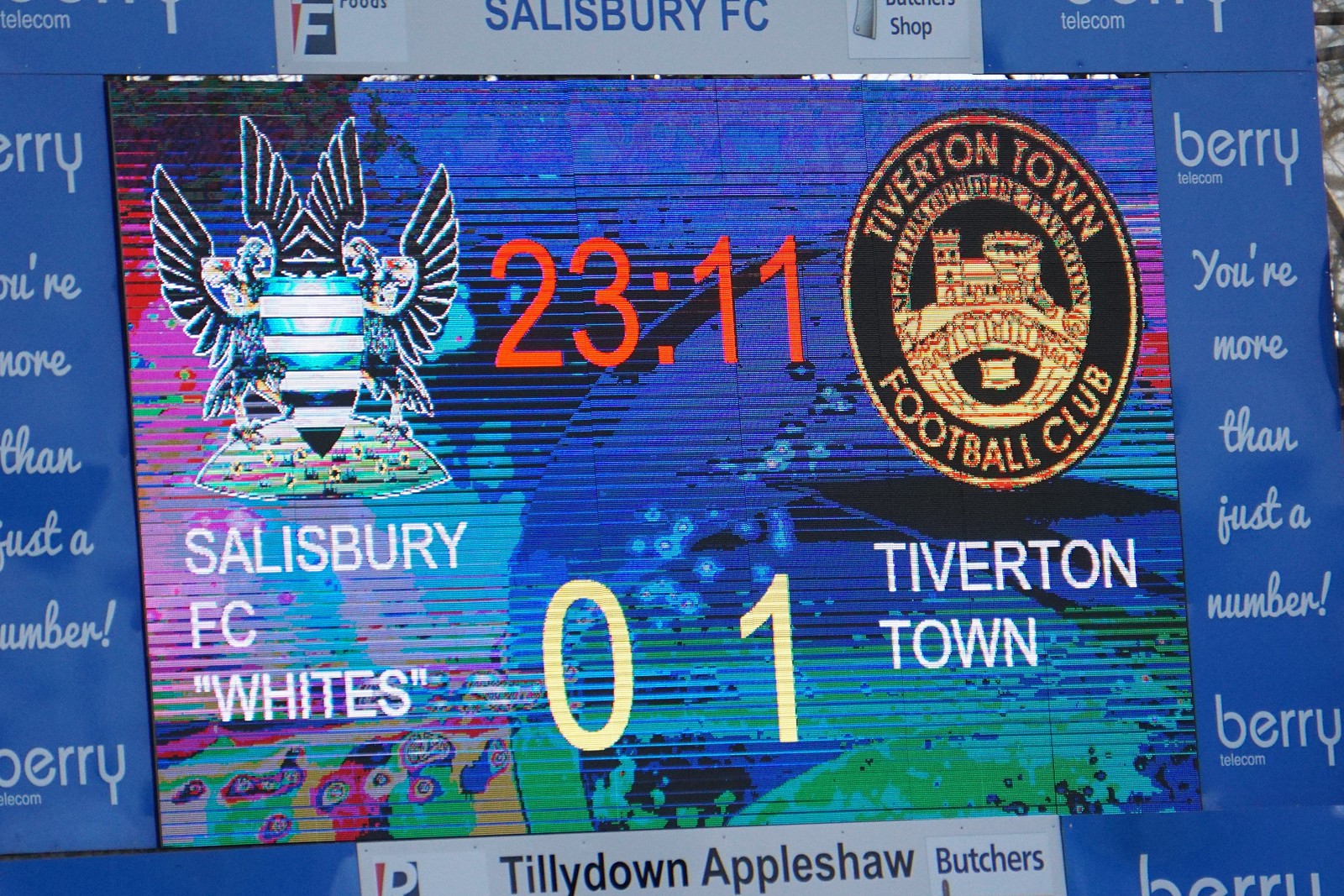The image captures a detailed view of a vibrant electronic scoreboard at a soccer match. The scoreboard prominently displays a match between Salisbury FC Whites and Tiverton Town Football Club. On the left side, the Salisbury FC logo, featuring two eagles facing each other with a shield icon in the center, is visible above the text "Salisbury FC Whites." On the right side, the Tiverton Town logo, which resembles an orange medallion with the words "Tiverton Town" and "Football Club" inscribed within it, is shown above "Tiverton Town" in white text.

Centrally positioned, the scoreboard indicates that the match is 23 minutes and 11 seconds in, with the current score showing Salisbury FC Whites 0 and Tiverton Town Football Club 1, as indicated by the yellow text below the red timer. In addition to the match details, the board features advertisements: "Barry Telecom - you're more than just a number" flanks the sides of the scoreboard, and "Tilly Down Appleshaw Butchers" appears below it. The entire scoreboard is mounted on a blue background, enhancing the clarity of the displayed information.